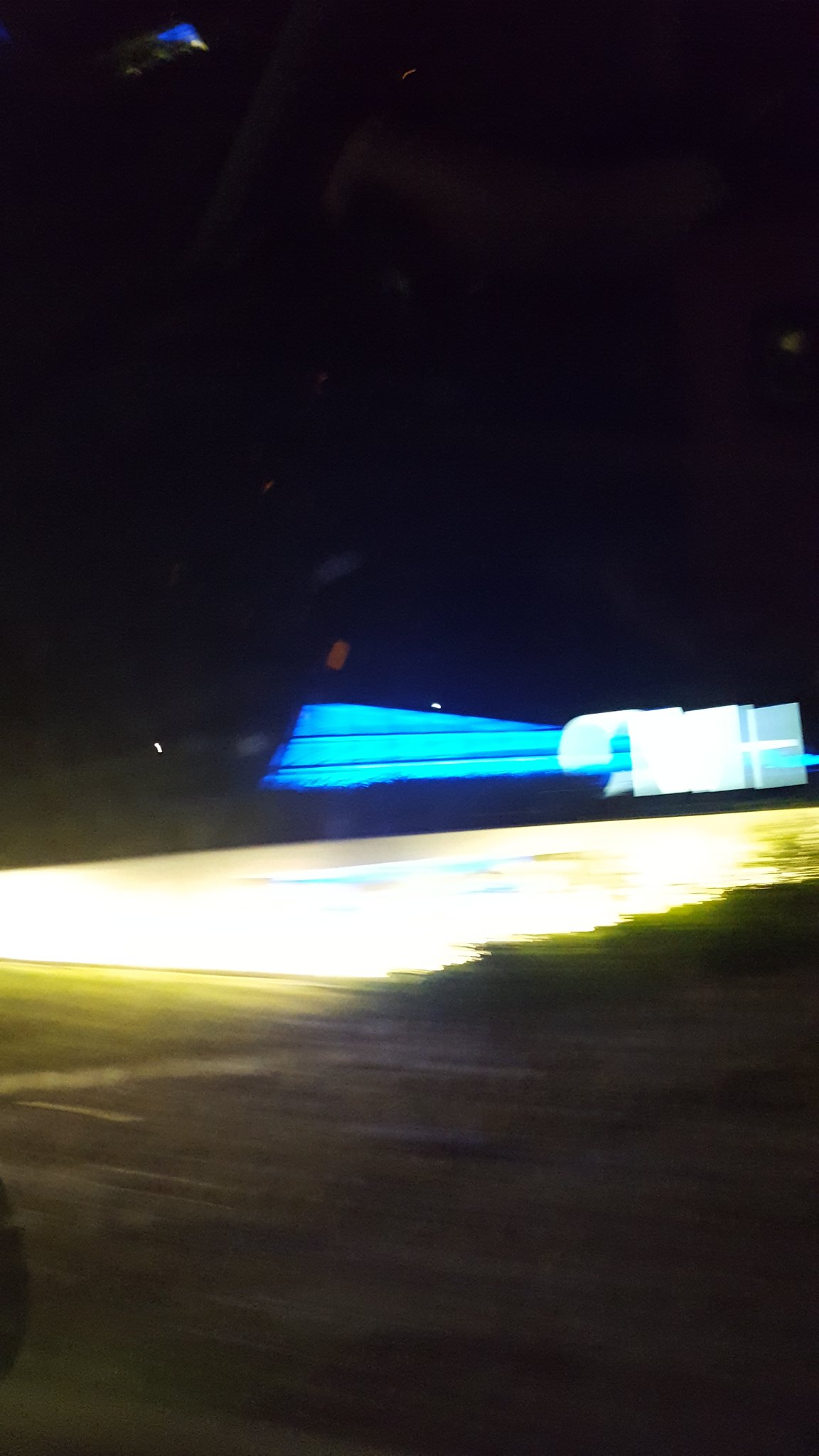This blurry nighttime photograph, oriented vertically, features a series of light streaks and contrasting colors against a dark sky. At the center of the image, a horizontal band of bright yellow light spans the width, casting a warm glow beneath it that gradually fades into a darker shade of yellow. This illuminated area below the yellow light transitions into an uneven, brownish-black sky. 

Above the central yellow band, and originating from the right side of the frame, is a streak of mixed blue and white light that cuts diagonally across the scene. This streak contrasts sharply with the blackness above it, likely indicating an artificial light source against the night sky. The stark blackness above the blue and white streak intensifies the fragmented and mysterious atmosphere of the photograph, further emphasized by the general out-of-focus nature of all light sources, making specific details indiscernible. The entire image presents an otherworldly and enigmatic visual narrative, emphasizing the juxtaposition of light against the void of night.